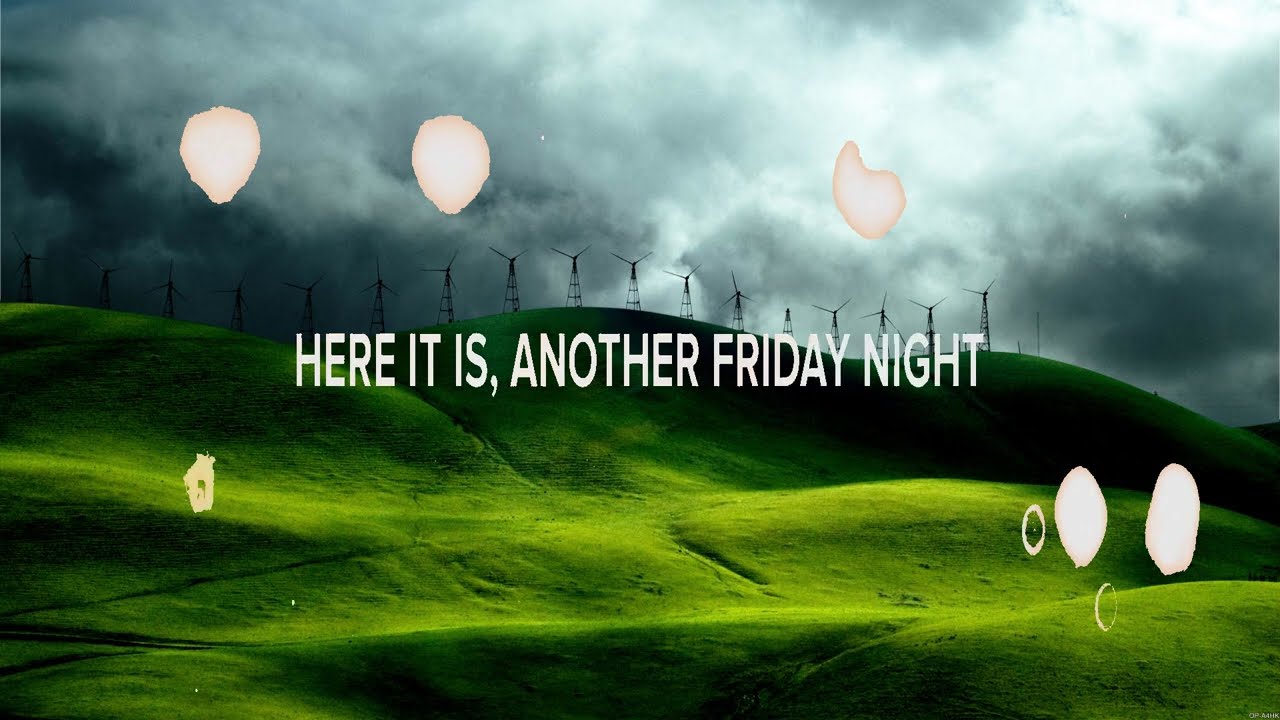The image depicts a vivid green rolling hill under a dark, stormy sky. The bright green fields cover the bottom half of the image, with numerous black windmills lining the horizon. Dominating the top half, the sky is filled with ominous gray and blackish-blue clouds, appearing thick and foreboding. Across the center, in bold white capital letters, the text reads "HERE IT IS, ANOTHER FRIDAY NIGHT." Scattered throughout the image are irregularly shaped pink and white splotches, resembling teardrops and oblong forms, adding an abstract and artistic touch. These elements, perhaps intentional design features, create a striking contrast with the natural landscape and add depth to the overall visual composition. The image’s style could be that of a visual graphic design, possibly an advertisement or an album cover, evoking a sense of solitude and reflection typical of a stormy Friday night.